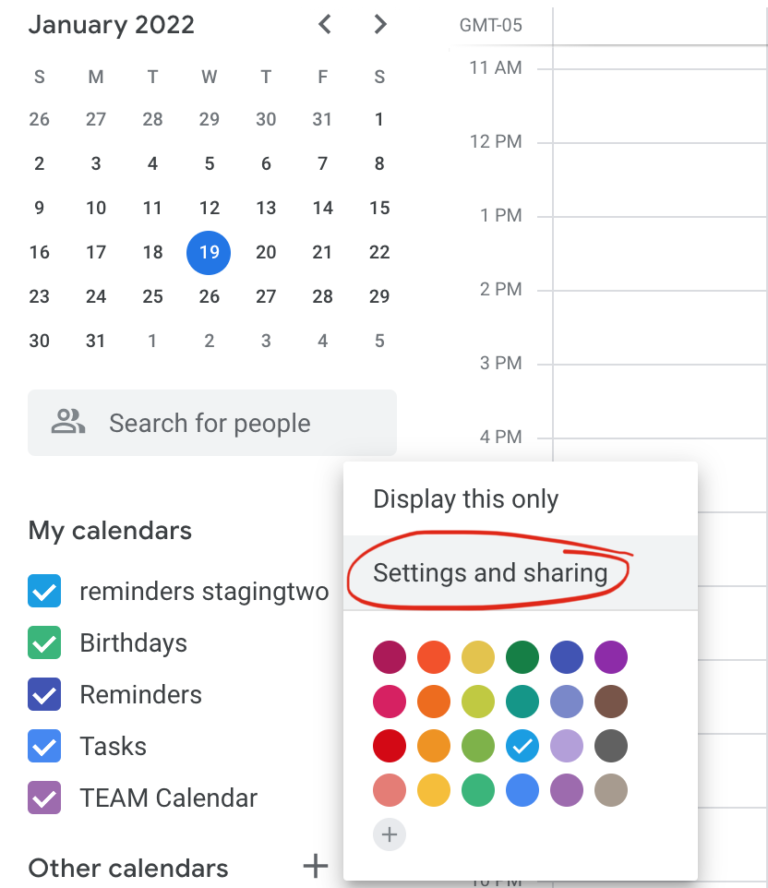In the image dated January 2022, the layout prominently features a calendar interface. At the top right, a small left-pointing arrow and a small right-pointing arrow are displayed, indicating navigation options. In light gray text, the timezone is marked as GMT-05. Below the header, the full month calendar is arranged starting from Sunday through to Saturday. The date Wednesday, January 19th is highlighted within a blue circle, drawing attention to this particular day.

Directly underneath the calendar, a search bar is present with placeholder text that reads "search for people." Below it, the section labeled "My calendars" shows five colored squares, each representing different categories: blue for Reminders, green for Birthdays, purple for Reminders, another shade of blue for Tasks, and a different shade of purple for Team calendar. Each square has a white check mark indicating their active status.

To the right of these squares, another icon is circled in red, labeled "Settings and sharing." Below this, there are four rows filled with circles in a variety of colors, including pink, red, orange, several shades of green, blue, purple, brown, and gray. This colorful array encompasses the different categories and settings within the calendar interface.